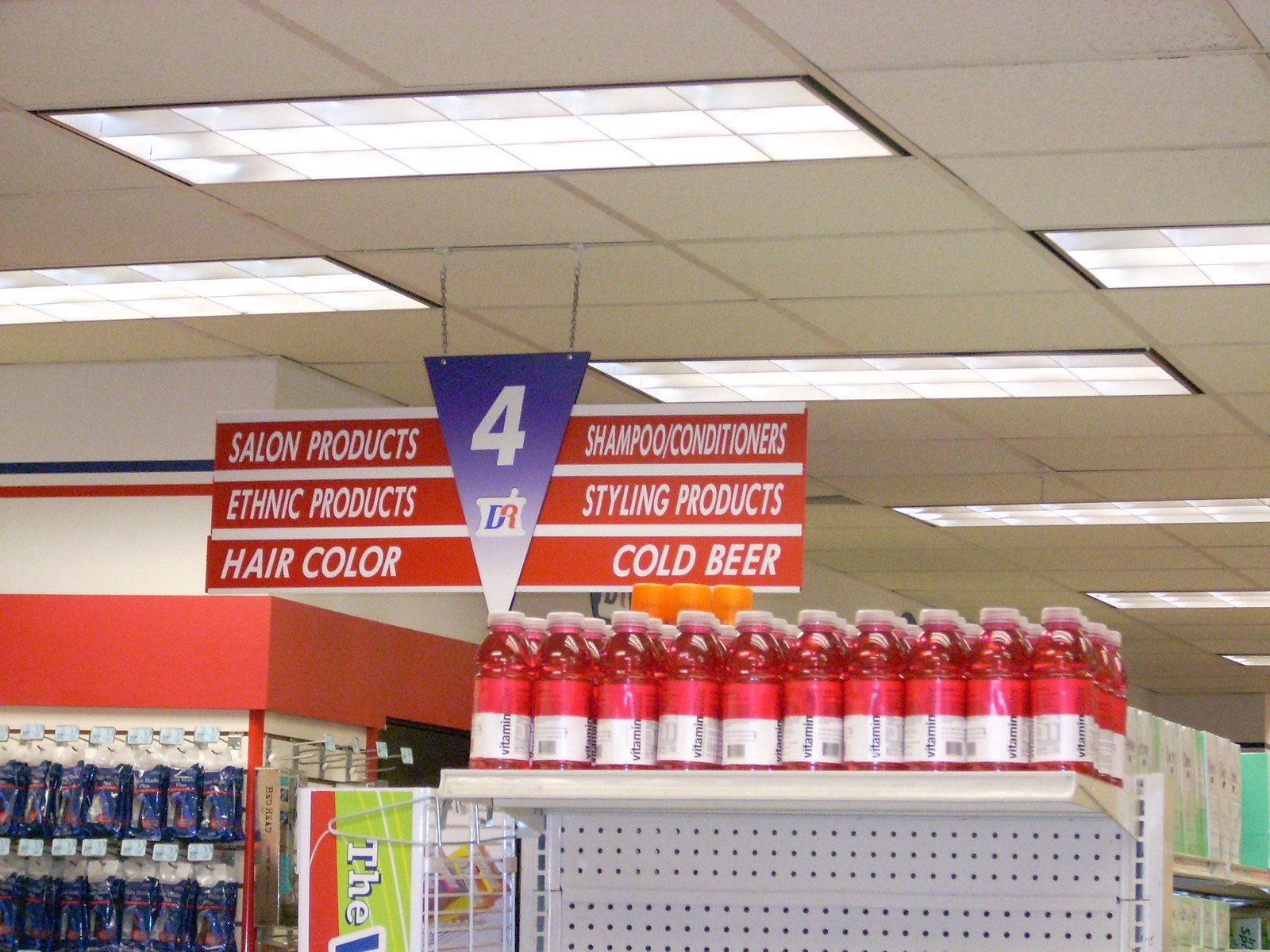In this photograph taken inside a Duane Reade pharmacy, the perspective is from the floor looking upward toward the ceiling, capturing a directional sign. In the foreground, there are clear plastic bottles of red Vitamin Water, each featuring a red and white label. The ceiling is paneled with recessed lights, providing ample illumination. 

Central to the image is a hanging purple pennant-style sign, marked with the number "4" in bold white font, accompanied by the Duane Reade (DR) logo below. The logo, an apothecary mortar and pestle design, is rendered in purple and red. The sign itself is bordered with red strips containing white text. On the left side: "Salon Products," "Ethnic Products," "Hair Color." On the right side: "Shampoo," "Conditioners," "Styling Products," "Cold Beer." 

In the background, the wall is decorated with Duane Reade's signature design — white, with purple and red stripes running across, aligning with the store's branding.